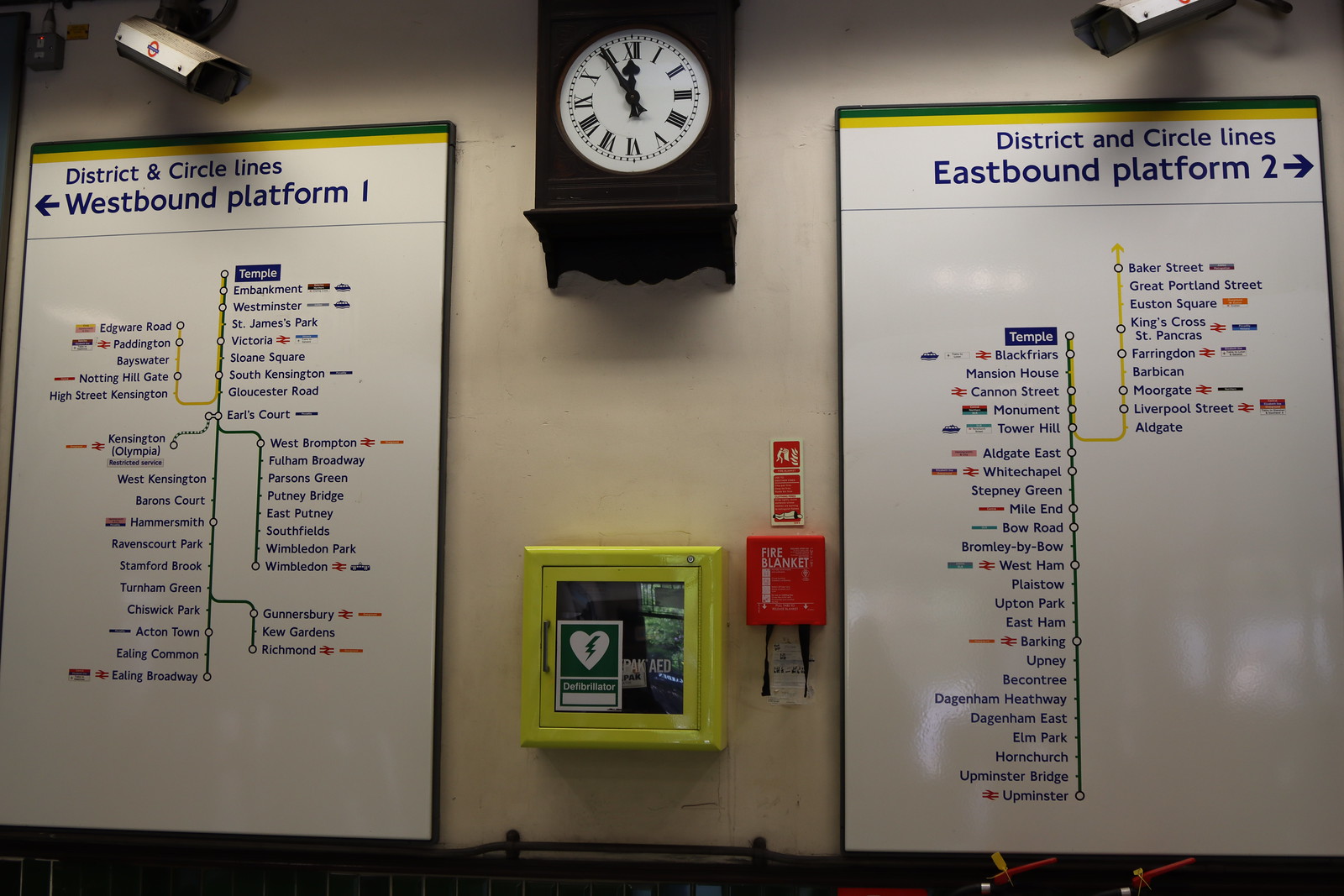This photograph depicts a metro train station showcasing two platforms, identified as Westbound Platform 1 and Eastbound Platform 2, which are part of the District and Circle Lines. Centrally located in the image is an old clock with Roman numerals and a white face, encased in a brown or black frame. Flanking the clock are two surveillance cameras, positioned in the top left and right corners of the photograph.

The left side features a white sign indicating "District and Circle Lines, Westbound Platform 1" with a left-pointing arrow, alongside a list of all the stops on that route. Similarly, to the right, another white sign reads "District and Circle Lines, Eastbound Platform 2," with a right-pointing arrow and a list of stops specific to that line. Both signs are marked with yellow and green lines, representing the respective lines on the subway map.

Beneath these signs, a red fire alarm is prominently installed, and there is a fire blanket emergency kit box mounted on the wall between the signs. The overall setting is a metro line or railway platform, captured in a photographic style that emphasizes the detailed layout of the station's informational signs, safety equipment, and surveillance features.